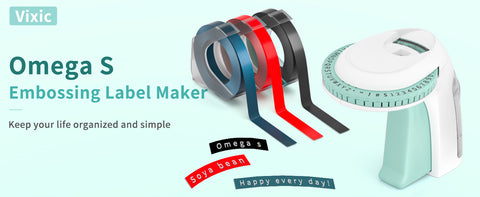The advertisement banner showcases the VIXIC Omega S Embossing Label Maker, designed to keep your life organized and simple. The banner has a light blue background with the product and its attachments displayed as if laid out on a surface. In the top left corner, a dark blue rectangle with white text reads "VIXIC," and beside it on the left, there's another dark blue text "Omega S," followed by lighter blue text "Embossing Label Maker" and smaller black text "Keep Your Life Organized and Simple." The focal point, a white and green label maker, is positioned on the right. To its left are three differently colored label strips—black, red, and teal—each with pre-printed sample texts. The black strip reads "Omegas," the red reads "Soyabean," and the blue reads "Happy Every Day!" These label strips also have matching cutouts below, demonstrating the printed labels. The entire setup is against the cohesive light blue background, enhancing the product's sleek and organized appeal.